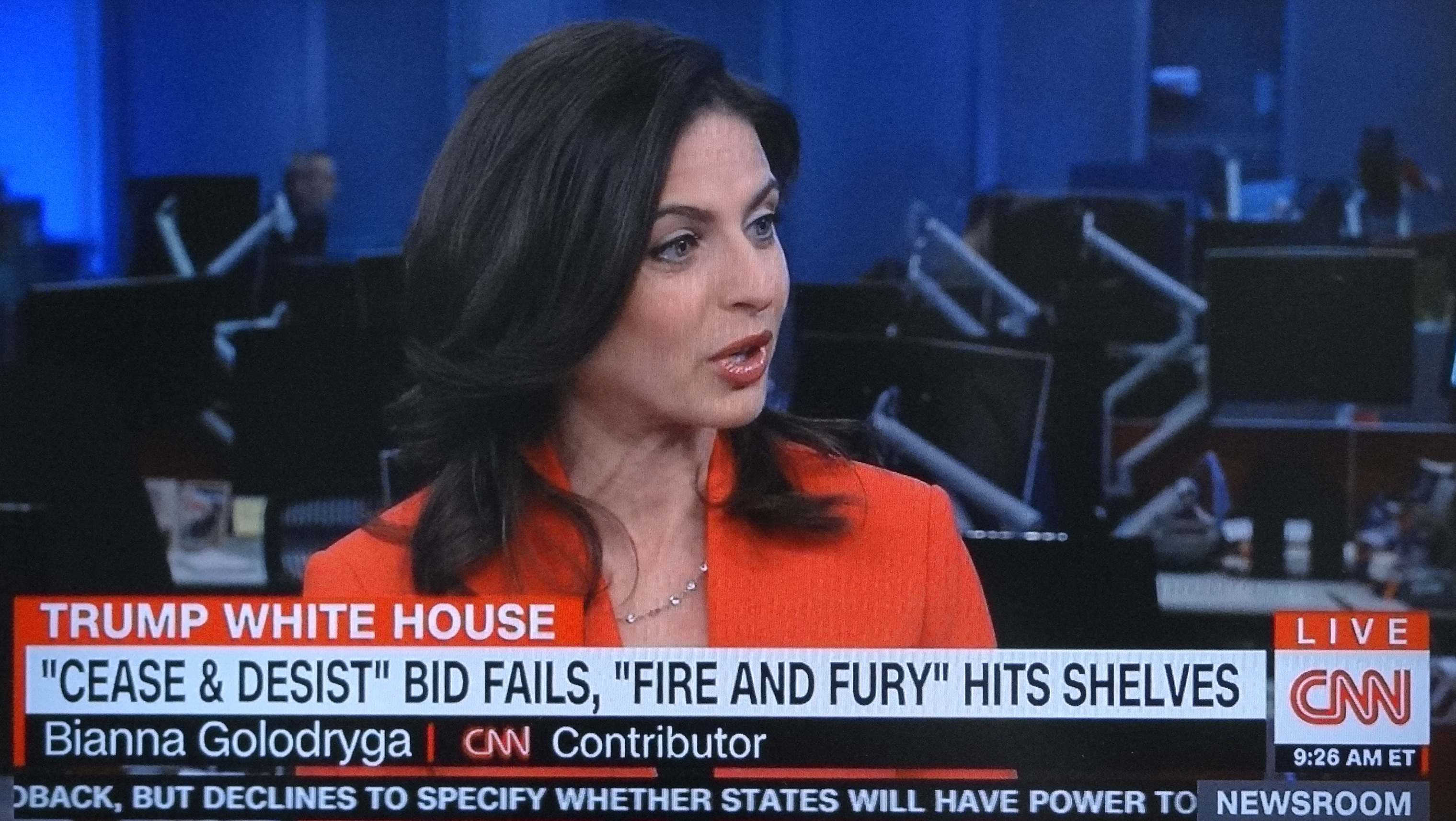This horizontally aligned rectangular image captures a screen cap from CNN at 9:26 a.m. ET. In the foreground, a female news anchor named Biana Golodryga, identified by an on-screen label, is speaking. She is wearing an orange suit-style jacket, complemented by a silver chain around her neck and pink lipstick. Her black, slightly curly hair extends just past her shoulders. She is facing towards the right, with her body oriented towards the viewer and her gaze directed to her left.

The lower left corner of the image details the following headlines: "Trump White House," "cease and desist bid fails," and "fire and fury hit shelves." Below these, the text displays her name and title, "Biana Golodryga, CNN Contributor." The lower right corner shows the CNN logo with "LIVE" in a red box above it.

In the background, there are multiple desks and large computer monitors, indicative of a busy newsroom. A few monitors are visible, with one additional person faintly discernible sitting at a desk on the distant left. The CNN ticker at the bottom of the screen partially reads, "declines to specify whether states will have the power to," though it is cut off. The overall setting seems to be a typical CNN newsroom with a mix of occupied and unoccupied desks.